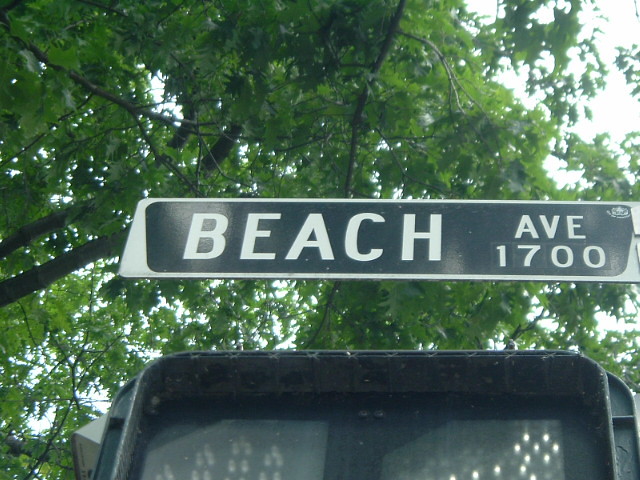This close-up photograph captures a street sign in sharp detail, surrounded by urban and natural elements. The street sign is a long rectangular shape with a black background and bold, white text that reads "BEACH" in all capital, sans-serif letters. To the right of this, the sign displays "AV" with "1700" positioned directly beneath it. The sign is bordered by a narrow white margin. 

The lower portion of the image reveals a glimpse of a rectangular pedestrian crosswalk signal with small, illuminated lights, although the message on the screen is partially obscured and unreadable due to the angle of the shot. 

The background features a dense array of tree branches adorned with lush green leaves, through which patches of the sky are visible. The sky has an overcast appearance, characterizing a bright, yet cloudy day. The angle of the photograph suggests it was taken from a low vantage point, looking upwards, providing an immersive perspective of the street sign amidst its surroundings.